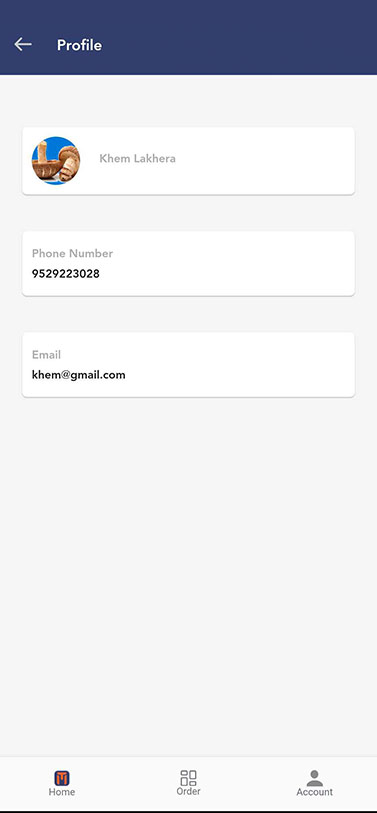This image is a screenshot of a user's cellphone displaying their profile page. At the top of the screen, the word "Profile" is prominently displayed in white lettering on a navy blue rectangular background, accompanied by a left-pointing arrow. Below the title, the user's name, "Khem Lakhera," is shown in large text with the name split into two lines: "K-H-E-M" on the first line and "L-A-K-E-H-E-R-A" on the second. An icon featuring mushrooms—one upside down and another laying on its side—is located next to the name, within an interactive bar button. 

Beneath the name, the phone number "952-922-3028" is listed, followed by the email address "kiem@google.com." The middle section of the profile page contains a large gray area that is notably blank. At the bottom of the screen, there are three navigation buttons: a home button with an icon embellished in orange, an order button symbolized by small rectangles, and an account button represented by the silhouette of a person.